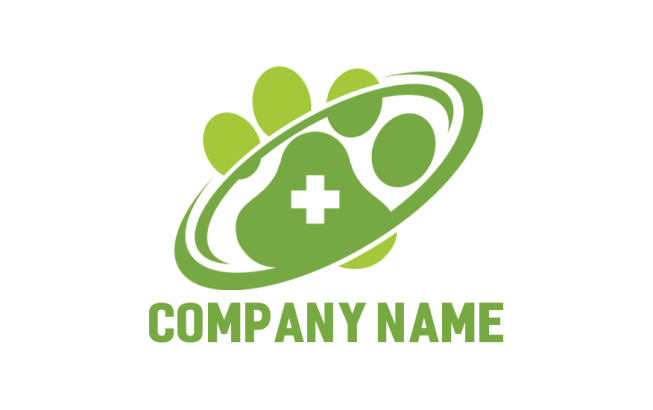The image features a graphic logo on a plain white background. Central to the design is a green paw print, depicted with a slightly darker green for the paw and a lighter green for the surrounding elements. The paw has a distinctive triangular shape, with four lumpy circles representing the animal's toes. At the center of the paw is a white medical cross, suggesting a healthcare or veterinary theme. Encircling the paw is a green, Frisbee-like swirl. Below this central emblem, the text "COMPANY NAME" is displayed in all caps, written in a green sans-serif font. The entire logo is two-dimensional and minimalist, primarily utilizing shades of green and white. This clean and straightforward design appears to be a logo template, potentially for an animal hospital or veterinary clinic.